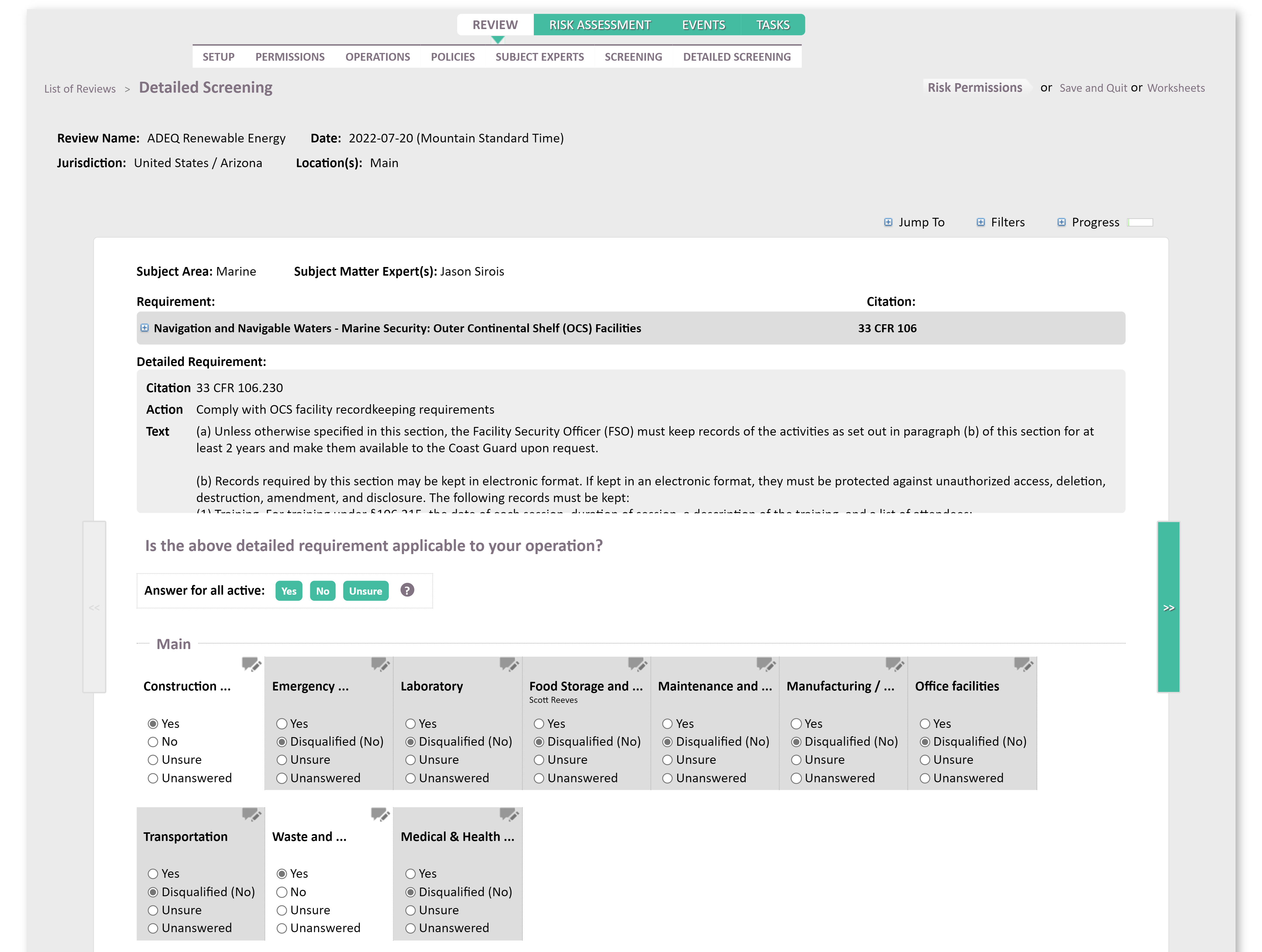**Detailed Caption:**

The webpage displayed appears to be part of a renewable energy program's comprehensive management system. At the top of the interface, there are navigation tabs labeled: "Review," "Risk Assessment," "Events," and "Tasks." Below these tabs, a secondary menu includes options such as "Setup," "Permissions," "Operations," "Policies," "Subject Experts," "Screening," and "Detailed Screening."

Directly under these sections, the page shifts to a particular function titled "List of Reviews," with a current focus on "Detailed Screening." In this detailed screening section, the "Review Name" is identified as "ADEQ Renewable Energy" with a noted date of July 20, 2022, in Mountain Standard Time. The "Jurisdiction" is indicated as "United States/Arizona," while the "Location" denotes "Maine."

The information continues under the headings "Subject Area: Marine" and "Subject Matter Expert: Jason Siraw." For "Requirement," the page lists multiple criteria including "Navigation In, Navigable Waters, Marine Security, Outer Continental Shelf (OCS) Facilities." Detailed requirements reference the legal citation "33 CFR 106.230."

Under the "Action" section, it specifies the compliance task: "Comply with OCS Facility Recordkeeping Requirements." The detailed text explains that, "Unless otherwise specified in this section, the Facility Security Officer must keep records of the activities as set out in paragraph B of this section for at least two hours and make them available to the Coast Guard upon request."

The page further prompts the user with the query, "Is the above detailed requirement applicable to your operation?" accompanied by options to answer "Yes," "No," or "Unsure" for all active requirements. A variety of qualifications follow, marked as applicable or not, such as "Construction, Emergency, Laboratory, Food Storage, Maintenance, Manufacturing, Office Facilities, Transportation, Waste, and Medical and Health," each currently selected as "Disqualified (no)."